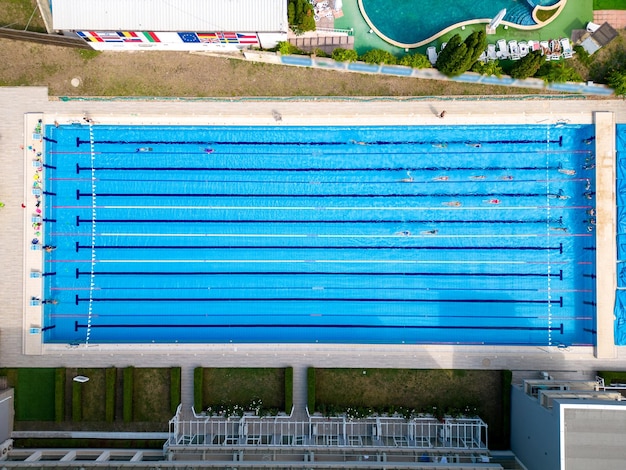The aerial view captures a vibrant outdoor scene centered around a large rectangular swimming pool used for competitive racing. The pool is filled with bright blue water and features eight distinct lanes marked by dark blue lines and white lane dividers. In the upper right corner of the pool, distant figures hint at activity, potentially a swim race. Surrounding the pool, the landscape transitions from well-kept green grass to sections of brown grass. Adjacent to the main pool, there is a uniquely shaped secondary pool, resembling a guitar or an oval, filled with vibrant blue water and bordered by a tan outline. White patio chairs are neatly arranged around this pool, adding to the organized ambiance. Prominent in the scene is a white building adorned with flags from various countries, emphasizing an international atmosphere. The building, with its white roof and walls, borders the main pool, while additional buildings and a spectator's gallery, greenery, and trees frame the entire area, enhancing the scenic and functional aspects of the setting.